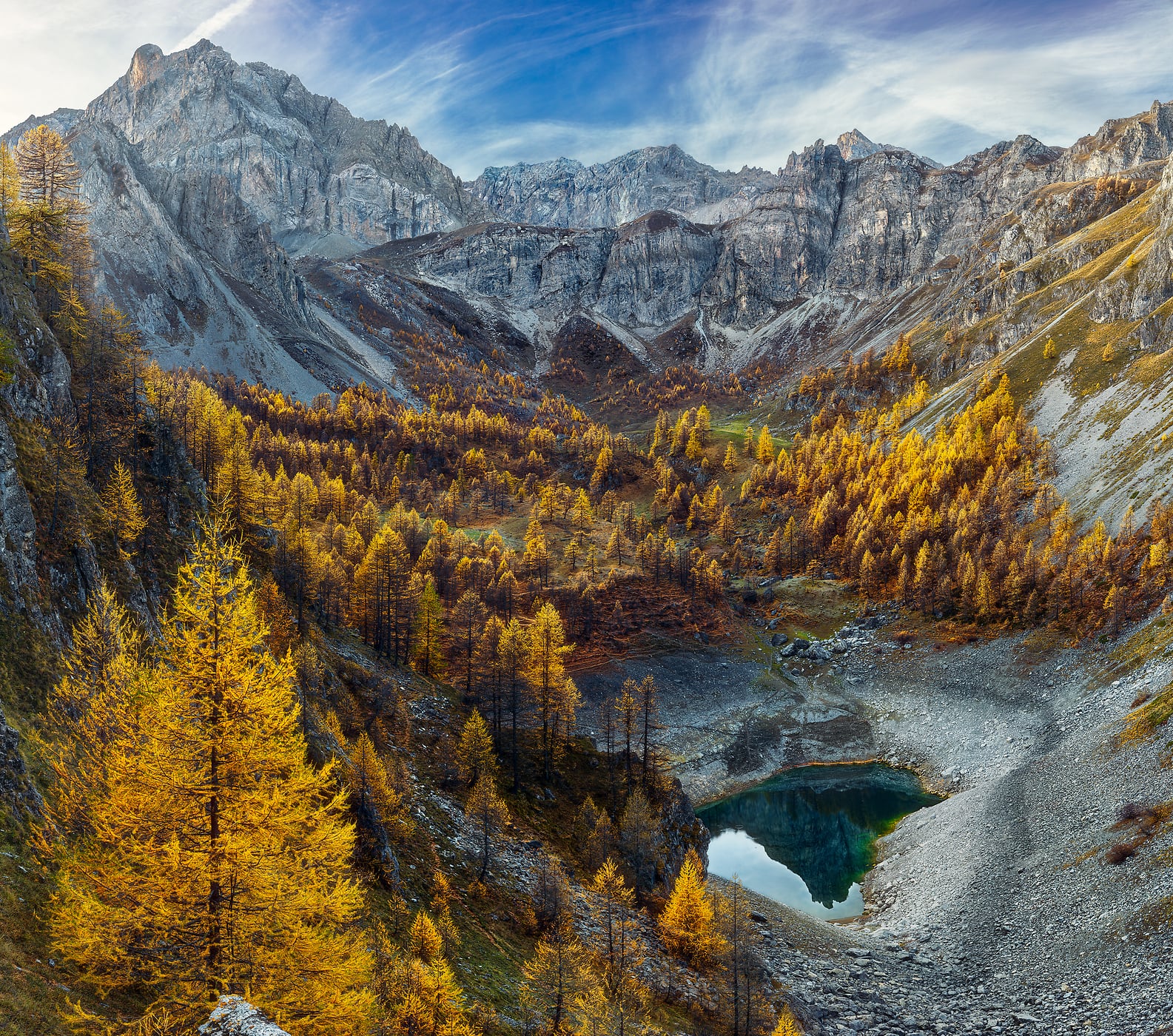The image captures a stunning and highly detailed scene of the wilderness, seemingly rendered or heavily edited for an enhanced effect. It is daylight, and the vibrant sky is painted with wispy white clouds. The central focus is a massive chasm surrounded by a rugged mountain range. The mountains in the distance exhibit a white tint on their peaks, suggesting a light snow cover, while the nearer slopes have no greenery, accented by deep red and brown shadows.

In the foreground, the terrain slopes down to reveal a rich forest of golden and brown trees, indicative of the fall season. These colorful trees encircle a small, crater-like body of water, which is a dark turquoise to greenish-blue hue—reflective and clear. The water, nestled within what looks like black dirt and rocky land, contrasts dramatically with the vivid foliage. The overall composition is both awe-inspiring and serene, capturing the intricate details and varying textures of this breathtaking natural landscape.